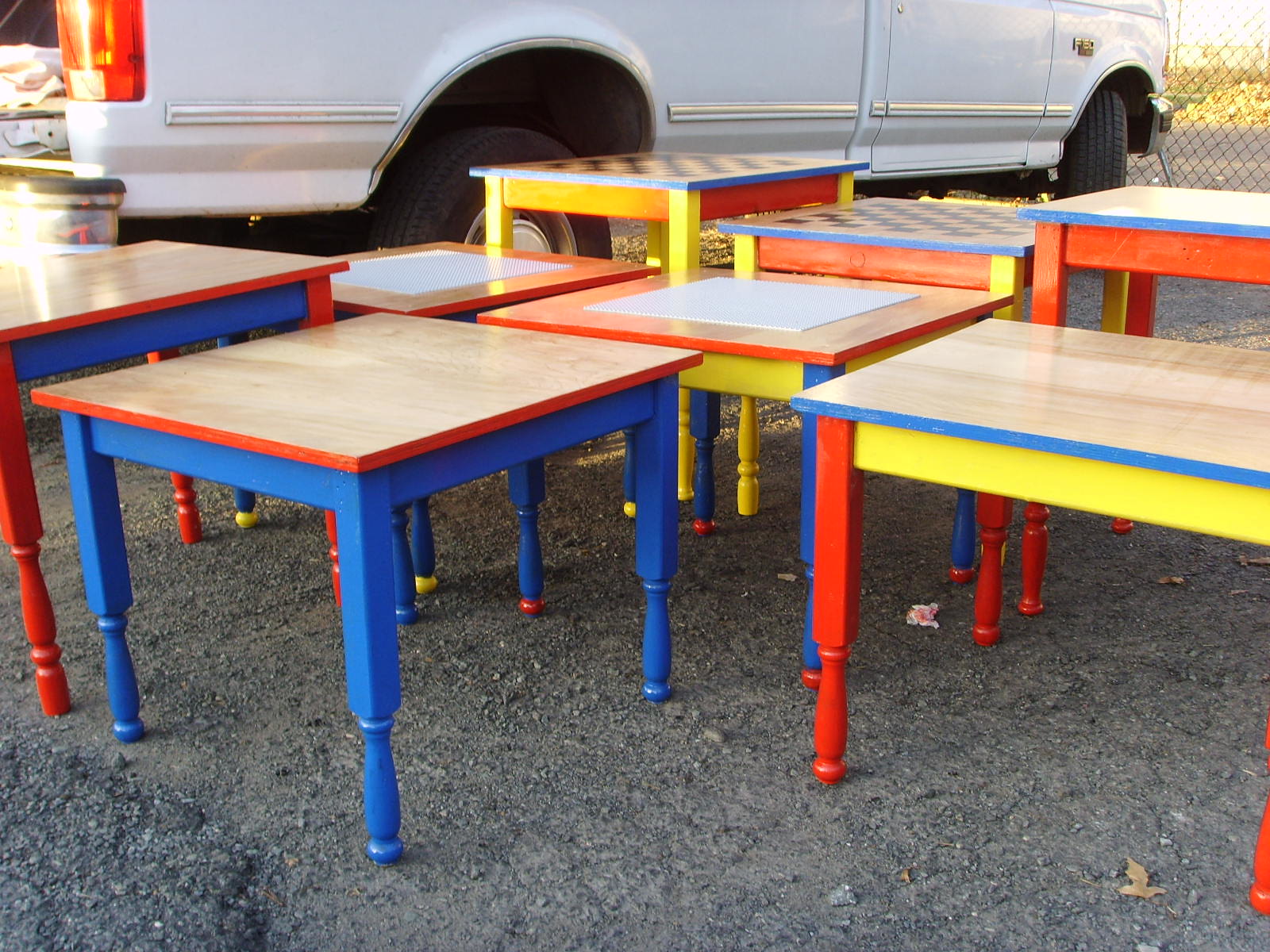The photograph, taken outdoors, depicts a collection of approximately eight small tables in vibrant primary colors, arranged on a rocky driveway. Most tables feature plain, sanded, and varnished light wood tops, while their legs and edges are vividly painted in red, yellow, and blue hues. Notably, two tables in the middle background proudly display checkerboard designs for playing checkers or chess. One prominent table in the foreground to the left contrasts its light wood top with a red-painted perimeter and a blue base with blue legs. Nearby, another table sports a rectangular shape, a light wood top, blue edging, red legs, and a yellow base. In the background, a white F-150 pickup truck is visible, oriented with its back to the left. A wire fence is notably positioned in front of this truck.